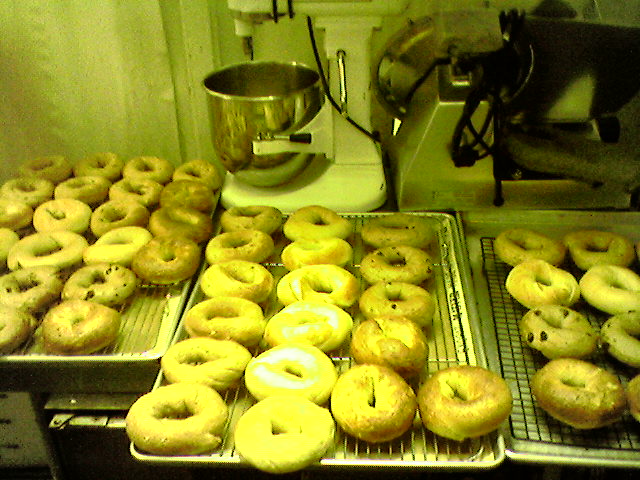This color snapshot captures the bustling interior of a commercial bakery kitchen, tinted with a yellowish-green hue suggestive of an older photograph. Central to the image are three pans of assorted bagels, neatly arranged on metal wire racks—two silver and one black. The bagels vary in type, with some appearing shiny and others featuring pieces of fruit, likely raisins. Their thick, substantial appearance hints at authentic New York-style bagels. Behind the racks, an imposing industrial-sized stand mixer with a large, deep stainless steel bowl stands out, though it currently lacks any attachments. Adjacent to it, a bread machine or possibly a meat slicer with a wrapped black cord contributes to the array of professional baking equipment cluttering the background. The overall scene exudes the meticulous yet homely atmosphere of a bakery, with a slight color distortion adding a nostalgic charm.